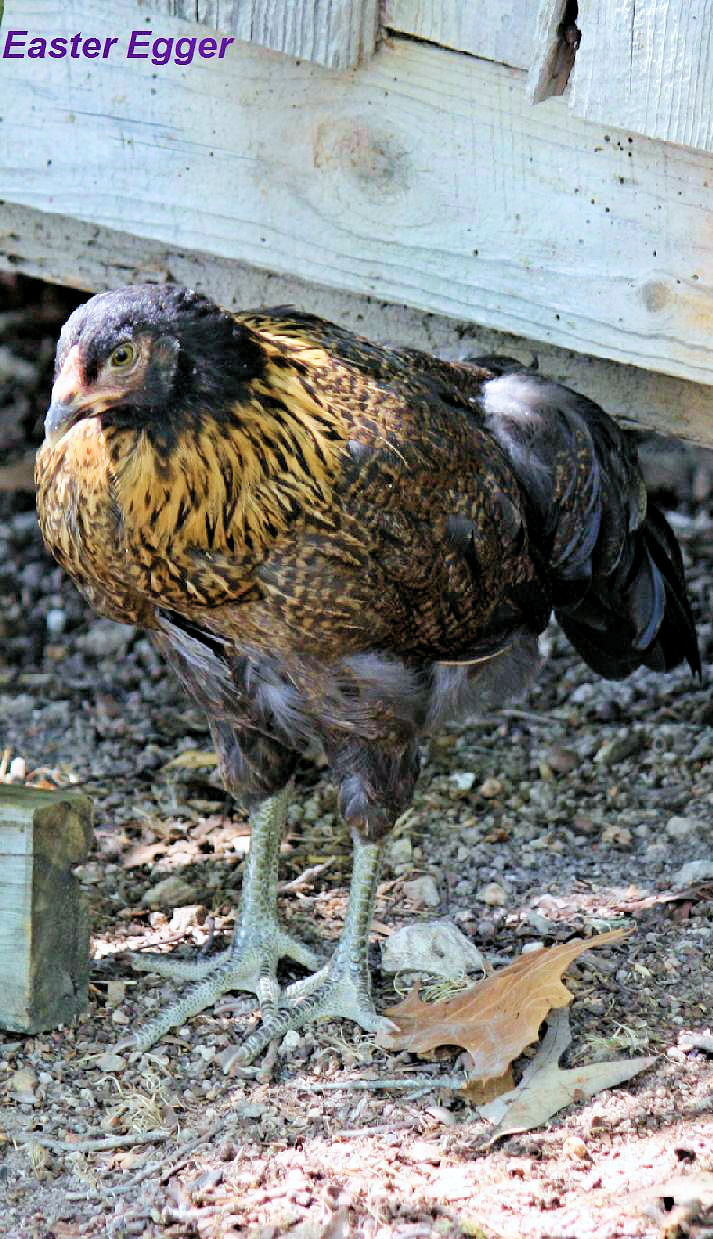The image depicts a rooster that is prominently featured in an outdoor setting on a bright day. The rooster, which is identified as an "Easter Egger" by purple lettering in the top left corner, showcases a striking array of colors and patterns. Its head is predominantly black with a red spot near the beak and green eyes. The neck area is adorned with yellow feathers trimmed in black, transitioning to orange and black on the chest. The body displays a mix of brown and dark brown-black feathers, while the tail feathers are dark blue and black. The rooster has long, greenish legs ending in sharp talons. It stands on a ground composed of dirt, rocks, leaves, and twigs, in front of a backdrop that includes a horizontally placed wooden plank and a vertically-aligned wooden fence, possibly part of a chicken coop. There is also another block of wood on the ground, contributing to the rustic, outdoor ambiance.